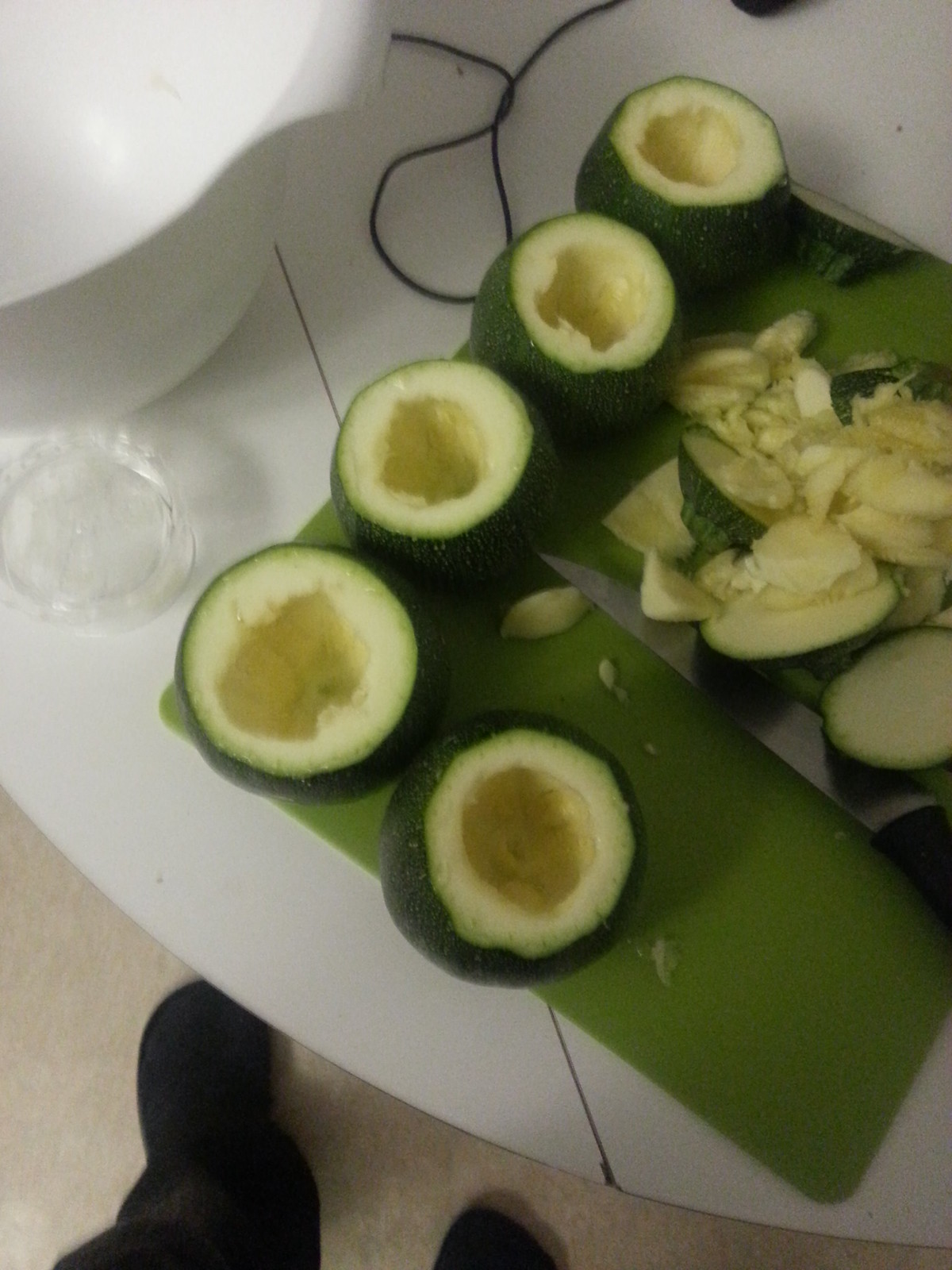This overhead photograph captures the edge of a white, round folding table set against what appears to be an off-white floor. Part of the image includes the black pant leg and shoe tip of a person standing by the table. Prominently placed on the table is a green cutting board topped with five round green vegetables, such as squatty gourds or hollowed-out squashes. The vegetables have had their tops removed and their insides scooped out, with the top pieces and flesh remnants arranged around them on the cutting board. A sharp metal knife with a black handle lies next to the vegetables. Besides this setup, a white pitcher, a glass of water, and a black cable—with its ends extending out of the frame—accentuate the scene.